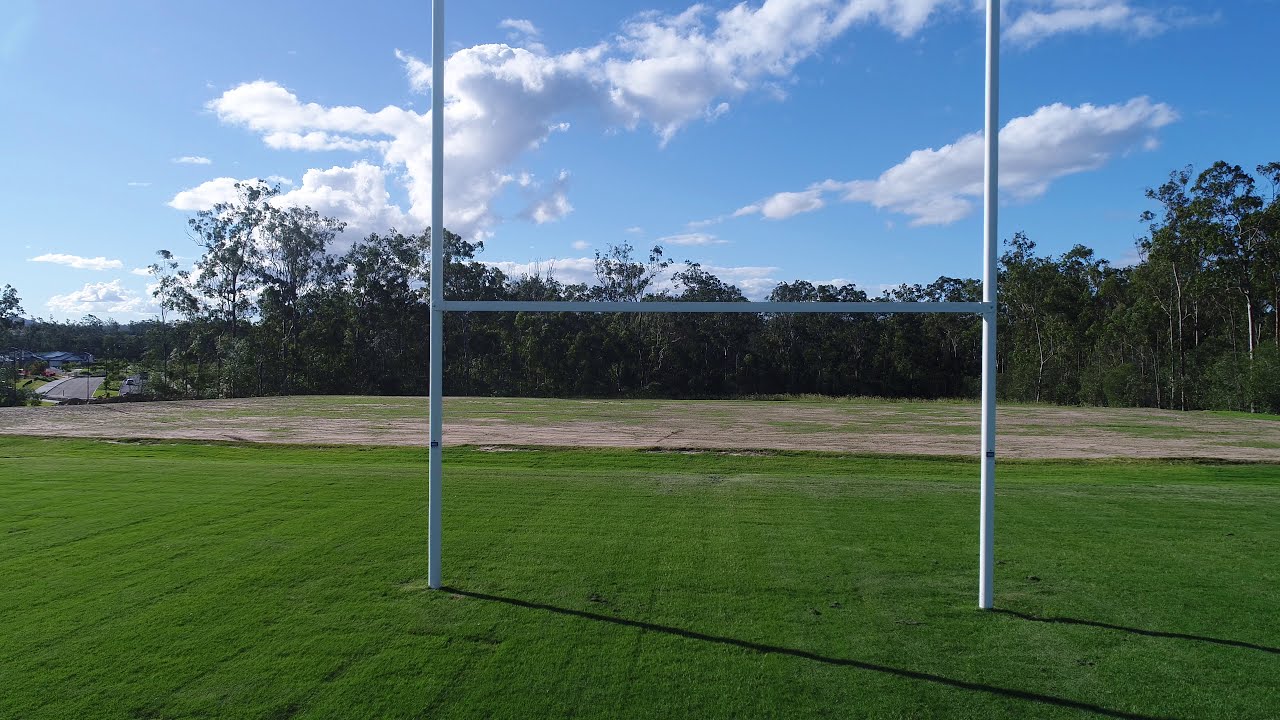The image is a landscape-oriented color photograph taken by a drone slightly above ground level, capturing a well-manicured grassy field. Centrally featured is a tall, white goalpost, resembling a large 'H' with two vertical poles extending from the ground and a crossbar in the middle, which can be used for sports such as football or pole vaulting practice. Shadows cast to the right of the goalposts indicate the presence of sunlight. In the background, the bright green grass transitions to patches of dirt and less vibrant grass. Beyond this, a horizontal row of tall green trees, possibly eucalyptus, lines the perimeter of the field. The sky above is a vivid blue dotted with white and gray puffy clouds, adding to the overall impression of a clear, pleasant day. The style of the image is photographic representationalism, emphasizing realism.